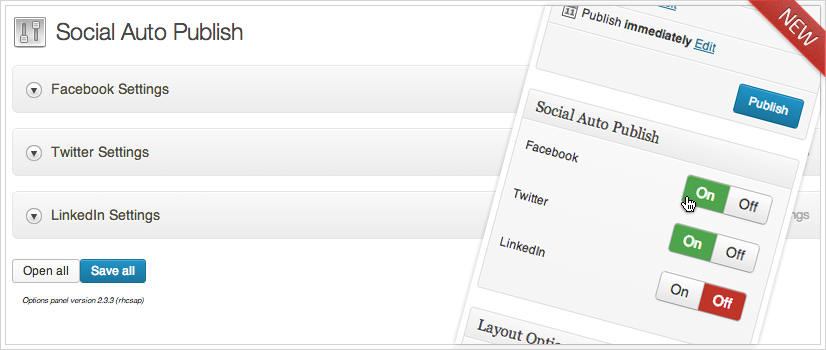This image is a screenshot of a website's settings interface. The background of the website is predominantly white, contributing to a clean and minimalistic look. 

On the right side of the screenshot, there is a graphic of a smartphone with sleek white bezels. The smartphone's screen displays a layout with gray squares and buttons. At the top of the smartphone's screen, the text "Publish Immediately" is prominently displayed, followed by a blue "Publish" button below it. The interface also features options for "Social Auto Publish" settings, listing platforms like Facebook, Twitter, and LinkedIn. Facebook and Twitter are toggled on, while LinkedIn is toggled off. 

A notable red banner with the word "NEW" in white font diagonally crosses the smartphone graphic, indicating a new feature or update.

To the left of the smartphone graphic, there is a vertical menu titled "Social Auto Publish." An icon resembling switches appears beside this title, enhancing the contextual understanding of the menu. Directly below this title, the menu lists three sections: "Facebook Settings," "Twitter Settings," and "LinkedIn Settings," each accompanied by a downward-pointing arrow that suggests expandable options.

At the bottom of the menu, two buttons are available: "Open All" and "Save All." The "Save All" button is highlighted in blue, emphasizing its importance for saving changes made in the settings.